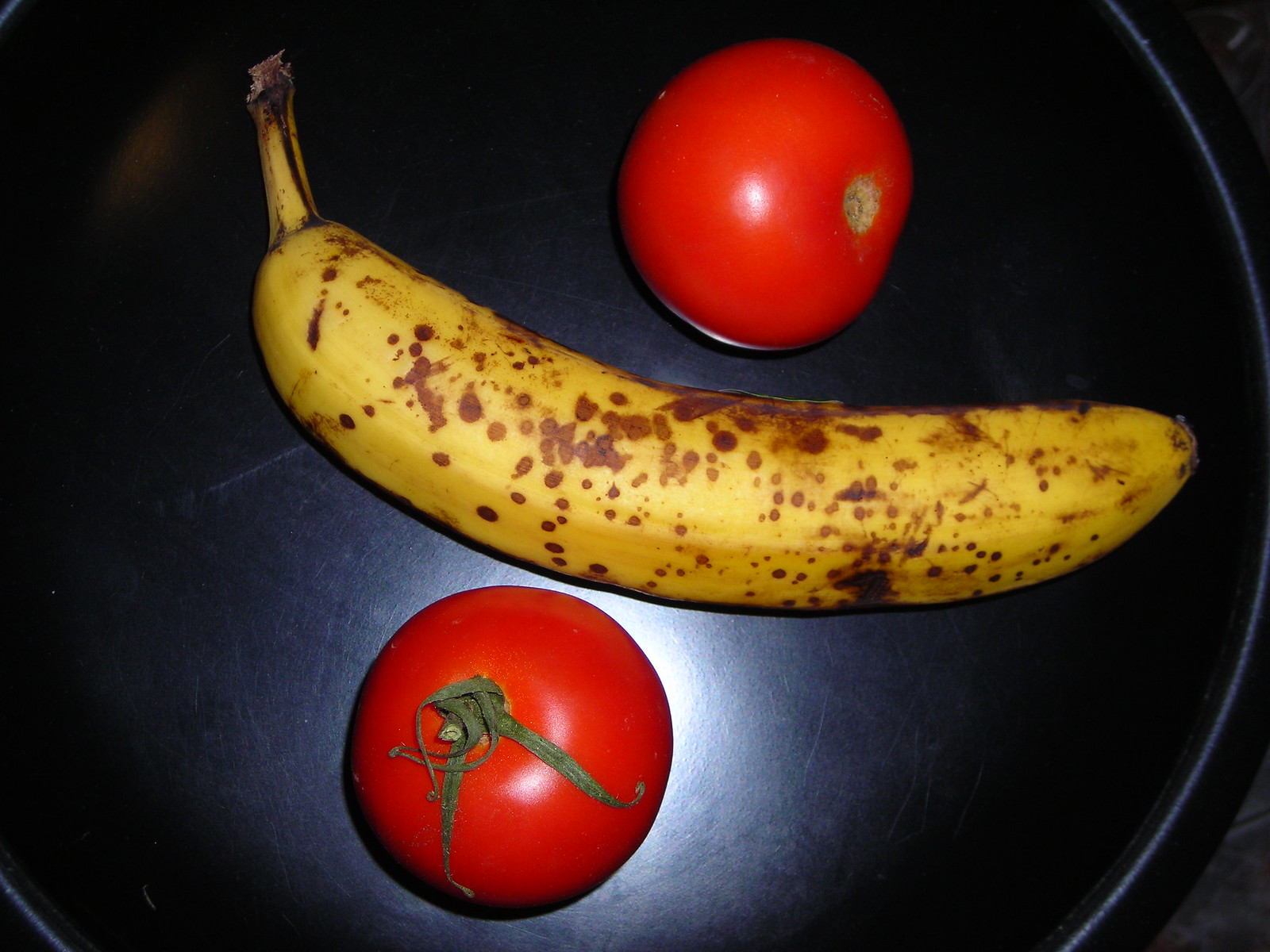In this photograph, a ripe banana and two vibrant red tomatoes are symmetrically arranged in a round, dark-colored bowl, which could be made of finely sanded plastic or painted wood. The banana, which is unpeeled and beginning to ripen, displays a striking contrast with its dappled appearance—approximately 65% of its peel is a rich yellow, interspersed with dark brown and black spots. Positioned horizontally in the center of the composition, the banana is flanked by the tomatoes—one on top and one on the bottom. One tomato prominently retains its green stalk, while the other is stalkless, enhancing the overall eye-catching simplicity and color contrast of the arrangement.